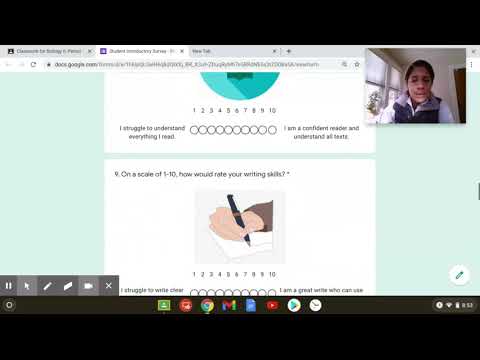This detailed screenshot depicts a Zoom or video chat screen with black bars running across the top and bottom, cropping the image. At the very top, a gray bar with multiple tabs open reveals the second tab as the active website. The main content of the screen shows a website with a seafoam green background and two white rectangles positioned vertically in the center. The lower rectangle features a prompt that reads "On a scale of 1 to 10, how would you rate your writing skills?" followed by a cartoon image of a hand holding a pen and a 1 to 10 rating scale. There's also a similar scale for reading skills, suggesting the content might be an aptitude test or an evaluation form. In the top right corner of the screen, an inset video feed shows a person, possibly a young man, looking down, presumably taking the test or tutorial. He wears a vest over a white shirt and is situated in a white room with windows visible to his left. The detailed setup hints at an interactive, possibly educational, online assessment.